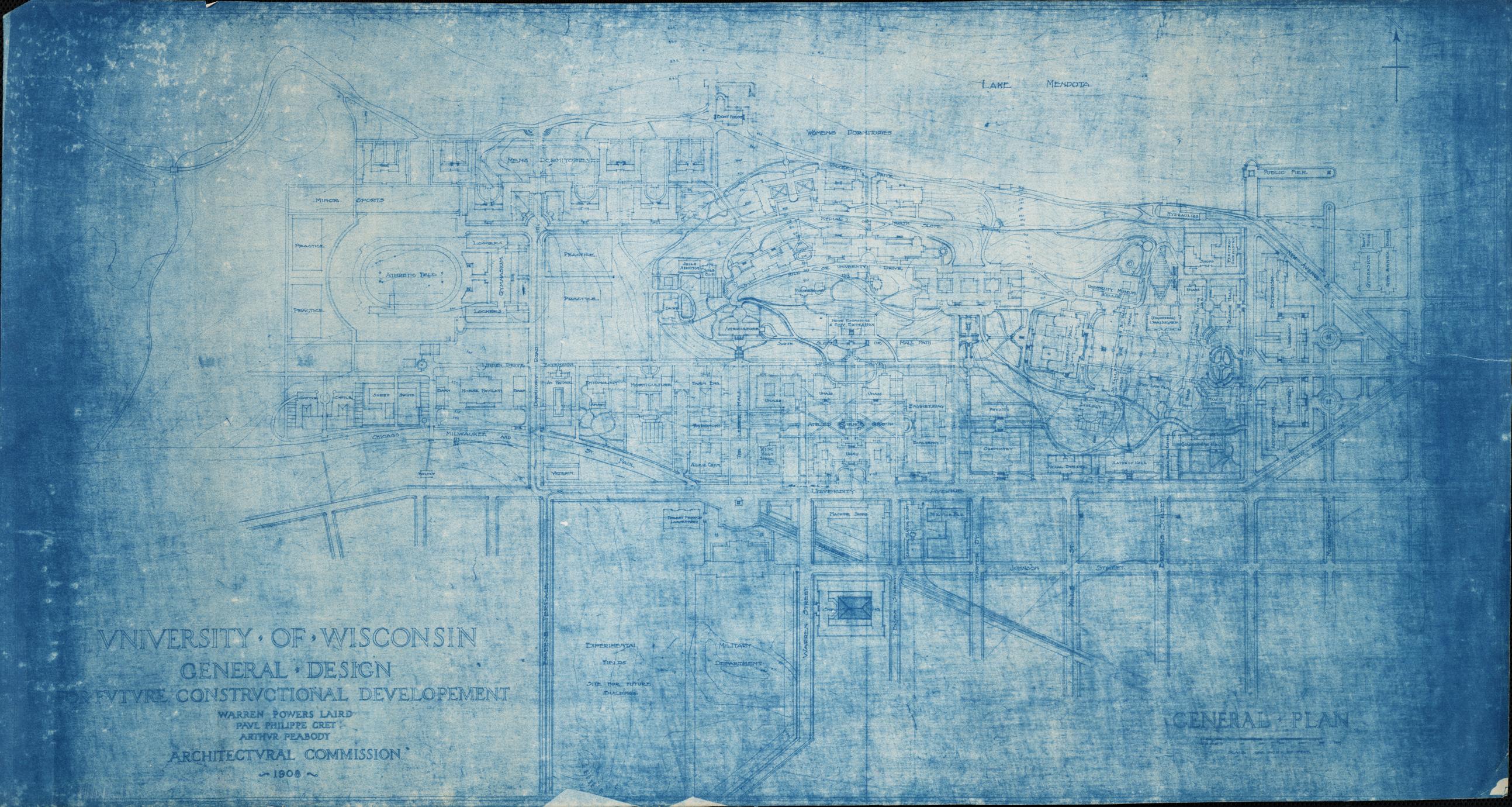In this vintage and intricate blueprint from 1908, the aged and highly detailed diagram showcases the architectural design of the University of Wisconsin campus. The blueprint, marked with blue tones and seemingly digitally altered from its original white background, has become somewhat faded and difficult to decipher over time. In the lower left corner, an inscription reads: "University of Wisconsin, General Design, Constructional Development, Architectural Commission, 1908."

The diagram meticulously outlines numerous buildings, rooms, and open ground spaces, suggesting a comprehensive layout of the campus. Although the individual names and functions of the buildings are indistinguishable due to the faded print, the layout includes what appears to be several roads or pathways traversing the campus. Despite the print's illegibility, the organizational structure is clear, indicative of a well-planned university campus.

In the lower right-hand corner, the words "General Plan" can be discerned, providing a clue to the purpose of this blueprint as a master plan for campus development. This historical document, despite its wear and low readability, offers a fascinating glimpse into the architectural ambitions and campus planning of the early 20th century.